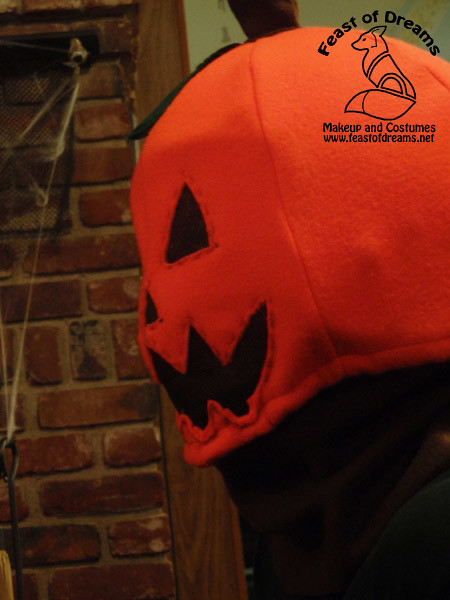The image is a vertically aligned, dark photograph that appears to feature a Halloween theme. The main focus is a jack-o'-lantern head made from a felt-like material, featuring stitched details around the eyes and a jagged mouth. The eyes and mouth are black, possibly made from a breathable fabric. This pumpkin head seems to be a mask or hood that covers an entire head, and it is worn by someone dressed in black, though the rest of their body is cut off by the bottom of the image.

The background shows an older red and brown brick wall, possibly part of a fireplace, with faux spider webs draped across it. The wall also has something, likely plants or vines, growing up it, indicating cold weather. Additionally, there are metal pokers at the base of the bricks.

In the top right corner of the image, there is a logo that reads "Feast of Dreams," accompanied by an illustration of a fox. Below the fox, the text "makeup and costumes, www.feastofdreams.net" is displayed.